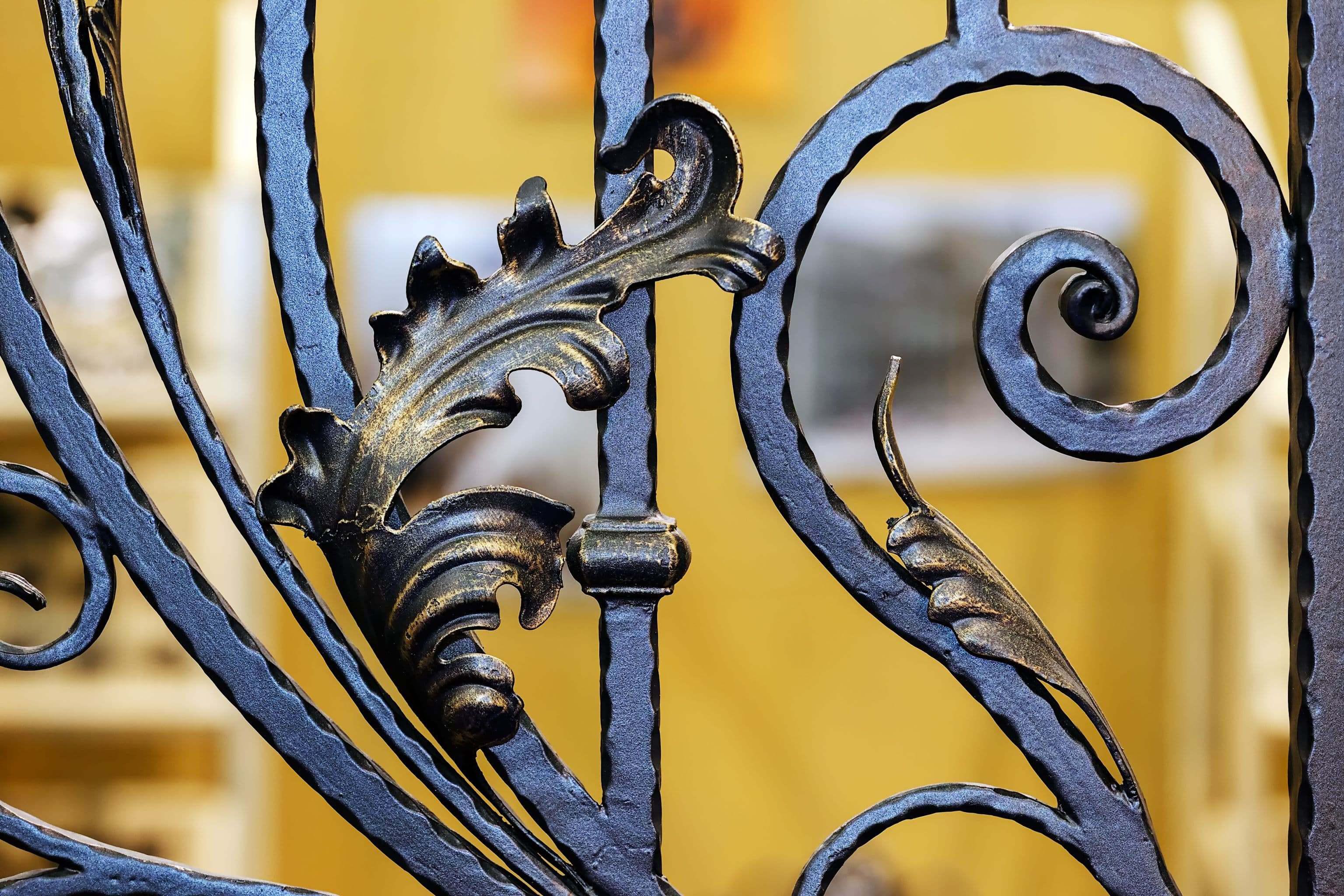This close-up photograph captures an ornate black wrought iron gate in intricate detail, with elements of gold leaf decorating its structure. The gate features a prominent swirled S-shape on the right-hand side, adorned with a gold leaf motif that ascends along the swirl. Additional details include three gracefully curved rods extending to the left, each embellished with delicate, gold leaf-like foliage. A golden-brown notched bar complements the overall design. The background reveals a blurred yellow building with white-framed windows and possibly a bookcase or other furnishings, drawing focus purely to the exquisite craftsmanship of the gate.